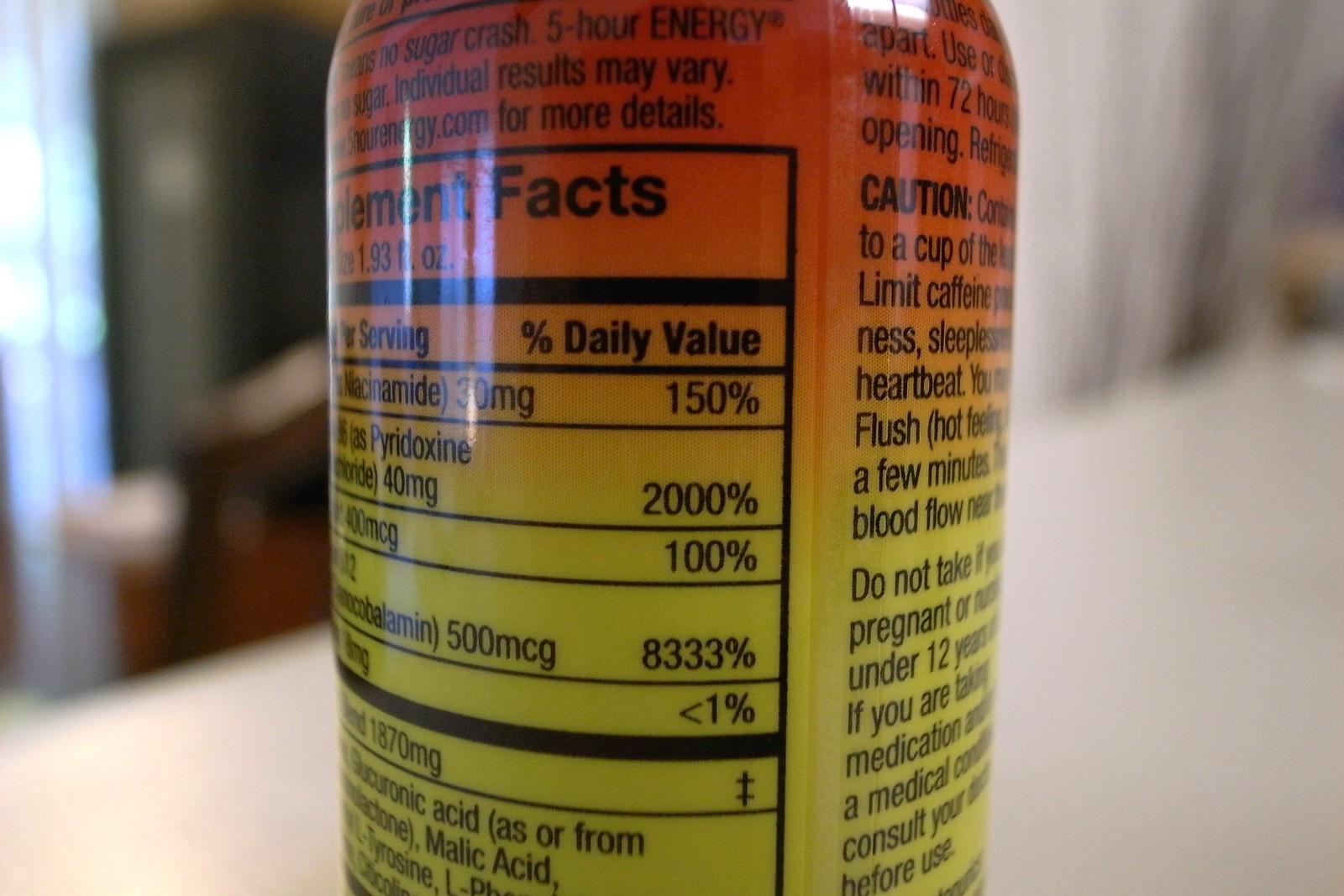The photograph showcases a portion of the back and side panel of a vitamin supplement bottle, potentially containing niacin or B vitamins. The label includes the nutrition facts, detailing the percentages of daily recommended values for various ingredients. The first ingredient provides 150% of the daily recommended value, while the second ingredient offers a staggering 2,000%. The third ingredient meets 100% of the daily recommended value, and the fourth ingredient supplies an extraordinary 8,333%. The fifth ingredient contributes less than 1% toward the daily recommended value. A dark line separates these details from another ingredient listed below, which notably lacks a percentage, likely because a recommended daily value has not been established for it.